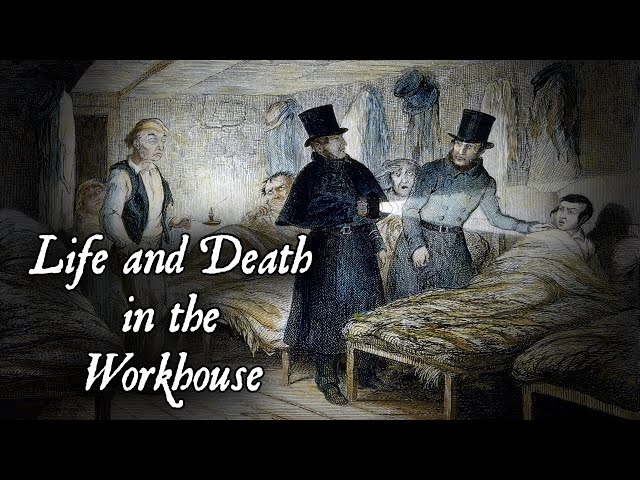The image appears to be a detailed, somber illustration evocative of a scene from a historical book. It prominently displays a distressed man lying in a bed, attempting to sit up. Surrounding him are two concerned men in ornate jackets and stovetop hats, reminiscent of Abraham Lincoln’s attire. One of these men shines a lantern on the bedridden figure, their expressions marked by worry. In the background, the cramped room reveals more beds occupied by other men, all sharing exaggerated facial features, suggesting artistic exaggeration. The atmosphere is dreary, with tightly packed cots lining the space and a sense of shared hardship. The image includes the textual caption "Life and Death in the Workhouse" in white font at the bottom left, underscoring the grim reality of the depicted scene. Additionally, the small room is filled with men dressed in long clothing, some with leather belts, indicating a communal living and working environment. This evocative artwork captures the harsh conditions and palpable tension within the workhouse.